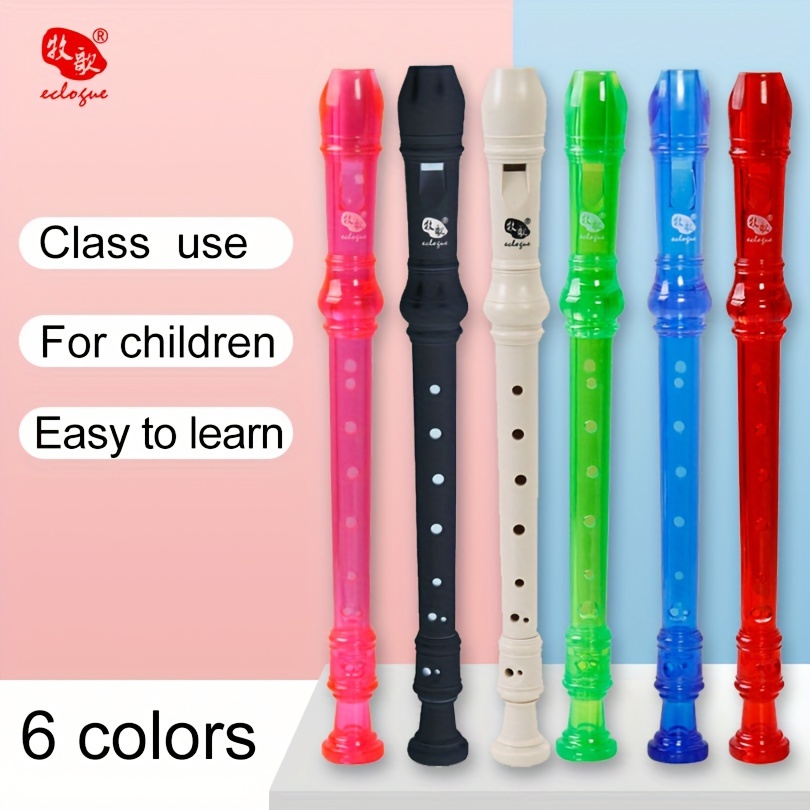This image is an advertisement for children's plastic recorders often used as a first musical instrument in elementary schools. The background comprises two-thirds pink on the left and one-third blue on the right, with six recorders lined up on a white platform in front of it. The six recorders, arranged from left to right, are transparent pink, black, white, transparent green, transparent blue, and transparent red. The top left corner features an unreadable red logo with Asian characters superimposed over the pink background. To the left, on the pink background, are three white banners containing black text that reads "Class use for children, easy to learn." At the bottom left, another black text on a white background states "Six colors." Each recorder prominently displays the company's logo on the mouthpiece.